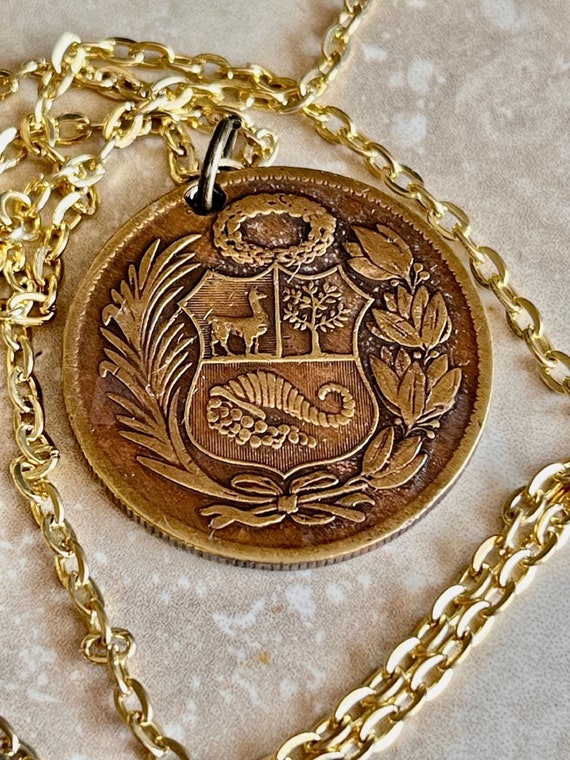This highly detailed vertical color photograph captures an intricately designed gold necklace with a medallion centerpiece. The chain is composed of bright, linked, 14-karat gold, neatly draped across a textured beige surface flecked with white specks, possibly a thick cloth or a tabletop. The medallion, which is a bronze-like color and slightly darker than the chain, features an elaborate design with two sets of leaves converging at the center, tied with a bow. Encircling the perimeter is a wreath-like pattern, possibly of wheat, adding to the antique aesthetic of the piece. In the middle of the medallion is a detailed crest split into sections: the upper left section depicts an alpaca or a llama, the upper right corner showcases a tree resembling the Tree of Life, and the bottom segment displays a horn of plenty, spilling fruit, likely grapes. The medallion is fastened to the gold chain by an oxidized, almost black clasp, and a silver connector, highlighting the age and mix of metals in this intriguing piece of jewelry.